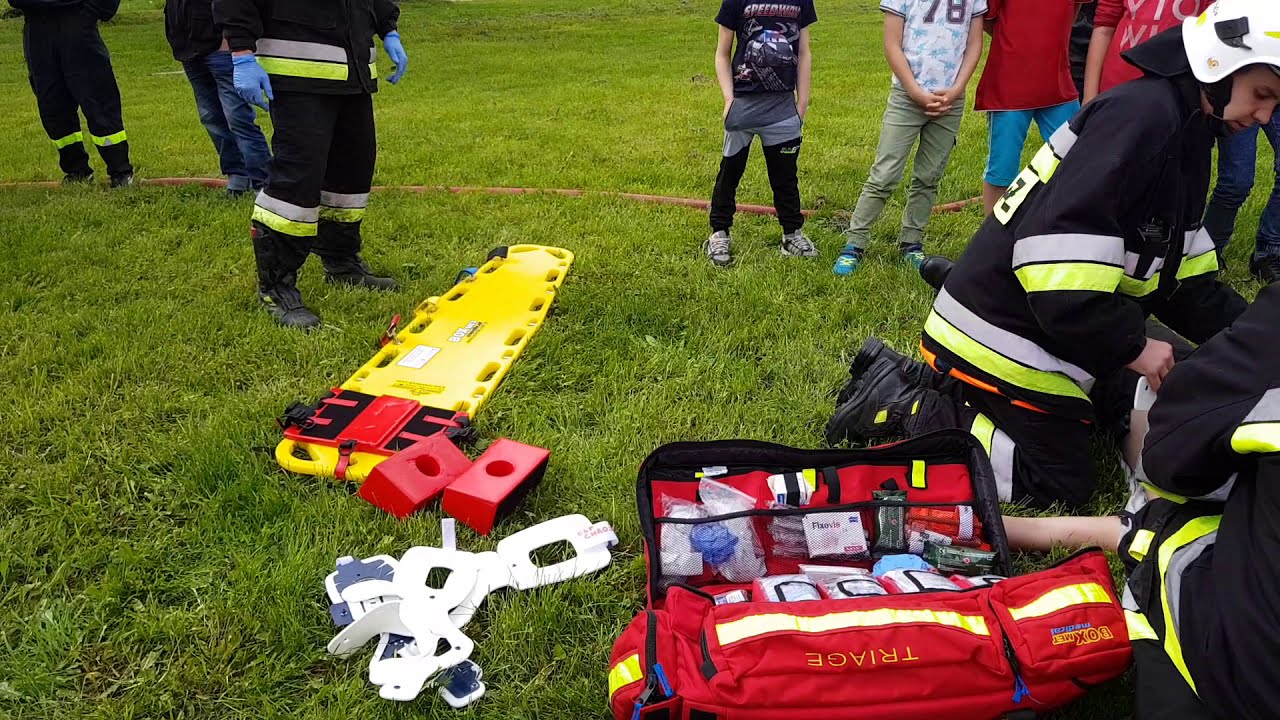The photograph captures a vivid scene of a first aid training demonstration, likely conducted for a neighborhood, with a particular emphasis on children as the audience. In the foreground, four paramedics dressed in black uniforms featuring reflective gray and neon yellow stripes around the elbows, back, and lower pant legs, are visibly engaged in a simulated resuscitation effort. One of the paramedics, identifiable by a white helmet, is actively attending to a person lying on the grass. Spread out on the ground are various pieces of medical equipment, including a large open triage bag, reminiscent of an airplane carry-on suitcase, revealing numerous medical tools, neck and knee braces, and other first aid supplies. Prominently placed nearby is a bright yellow stretcher equipped with orange neck supports, designed for spinal injuries. Surrounding the paramedics, a group of children—discernible mostly from the chest down and clad in casual t-shirts—observe attentively, underscoring the educational aspect of the demonstration. The scene is a well-coordinated blend of practical training and community engagement.